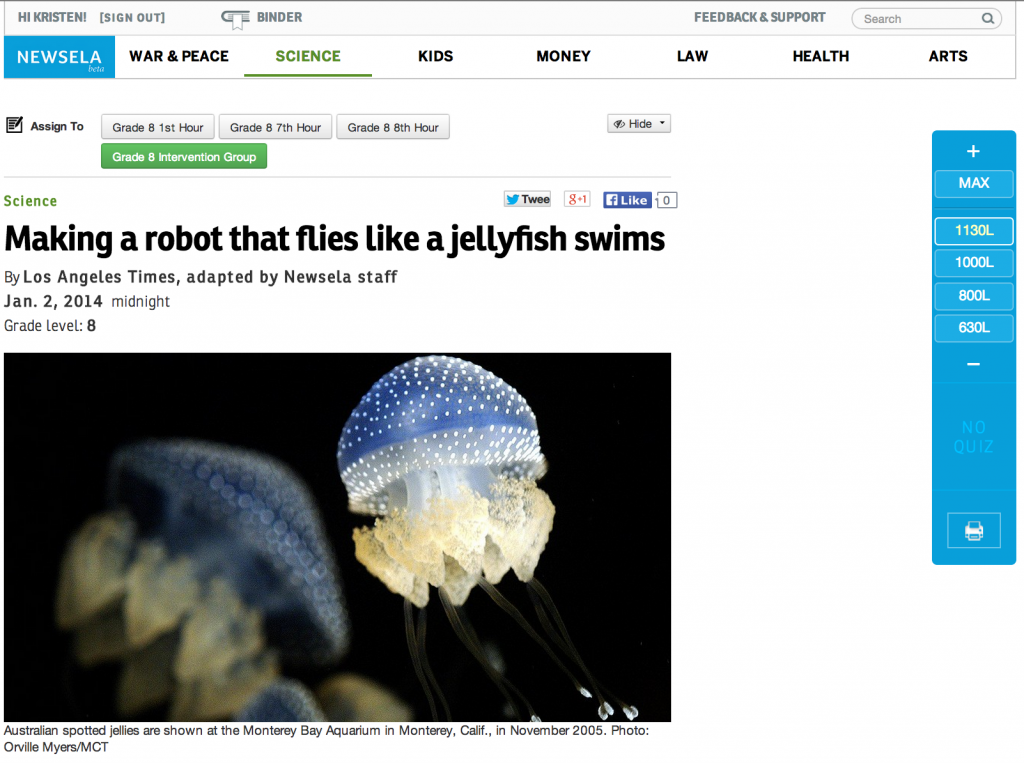This image appears to be a screenshot from an educational website interface designed for teachers. 

In the upper left corner, there are several options: "Hi Kristen," "Sign Out," "Binder," "Feedback and Support," and a search button. Below these, a navigation bar includes several tabs: "News," "illa," "War and Peace," "Signs," which is highlighted in green, "Kids," "Money," "Law," "Health," and "Arts." There is also a search box present.

The content on the page is focused on assignments for Grade 8. Specific times, such as "1 hour," "7 hours," and "8 hours," are listed, although their exact meaning is unclear. The "Grade 8 Intervention Group" appears to be the selected category.

A headline beneath these tabs reads, "Making a Robot That Flies Like a Jellyfish Swims," by the Los Angeles Times, adapted by Newsley Staff on January 2, 2014, at midnight. The content is indicated to be suitable for Grade Level 8.

The image accompanying this headline depicts a jellyfish resembling a blue toadstool with white spots and diamond-shaped yellow appendages. Another blurred jellyfish is visible on the left side of the image. The caption below the image reads, "Australian spotted jellies are shown at the Monterey Bay Aquarium in Monterey, Calif., on November 20, 2005. Photo by Anvil Myers MCT."

On the right side of the page, there is a vertical blue bar with white text that includes options such as "max" and several lexile levels ranging from 1130L to 630L. Additional buttons include a "minus" button, a greyed-out "no quiz" button, and a printer button at the bottom.

The overall layout and elements suggest that this website allows teachers to assign and manage educational content for their classes.